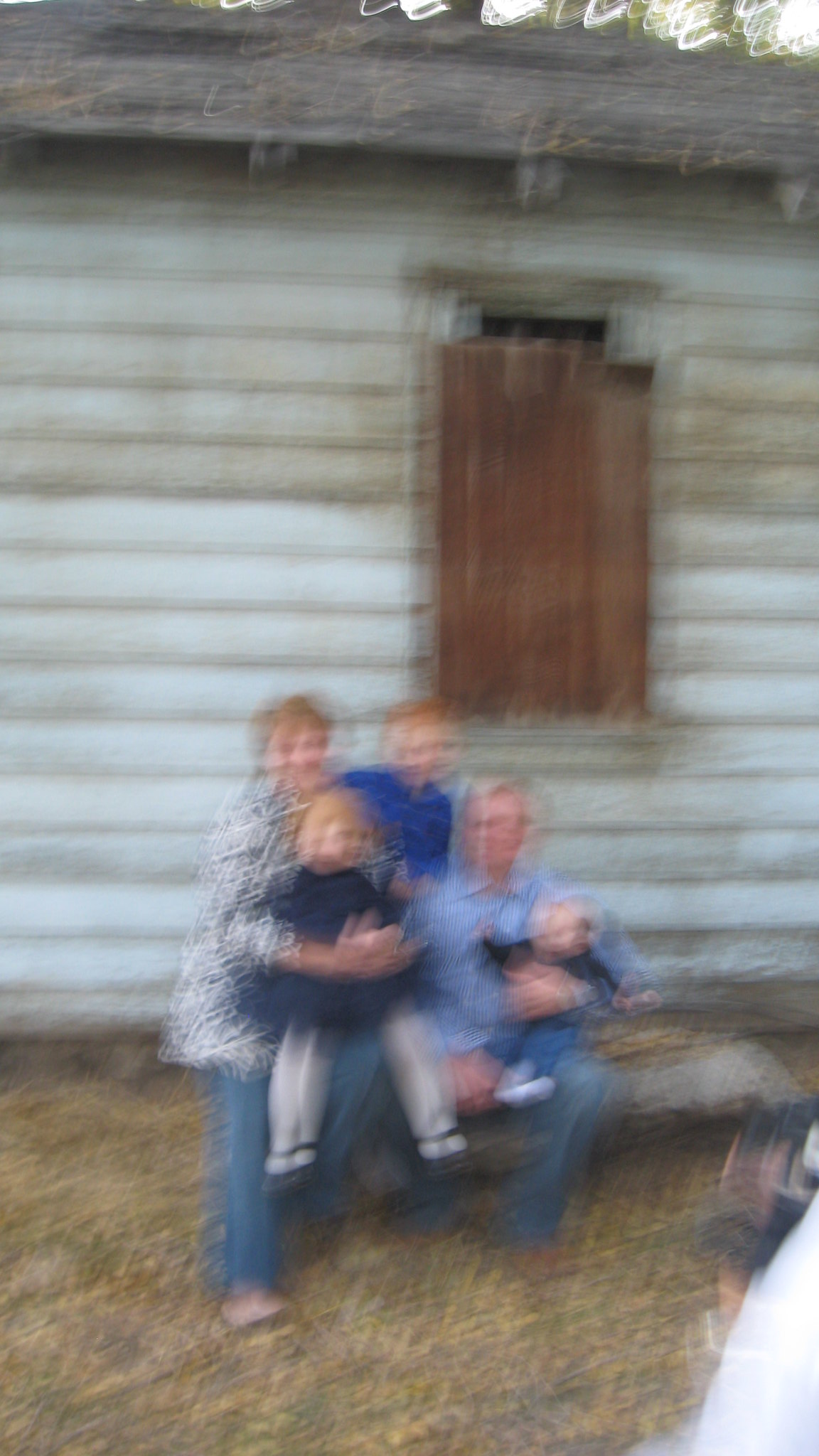A blurry photograph captures a family seated in front of an old, worn-down white building. The building’s roof is covered in grayish-black shingles and its siding, though originally white, is now marked with dingy streaks of black and dark brown. Behind the family, a window is boarded up with brown wooden planks.

In the foreground, the family sits on what appears to be a gray object, with green and yellow grass at their feet. On the left, a woman with blonde hair, wearing a dark blue dress, holds a small child on her leg. Next to her, a young boy with red hair sports a light blue shirt. On the right, a male figure is seated, holding a very small infant in his arms. Despite the image’s lack of clarity, the scene exudes a sense of rustic charm and intimate family bonding.